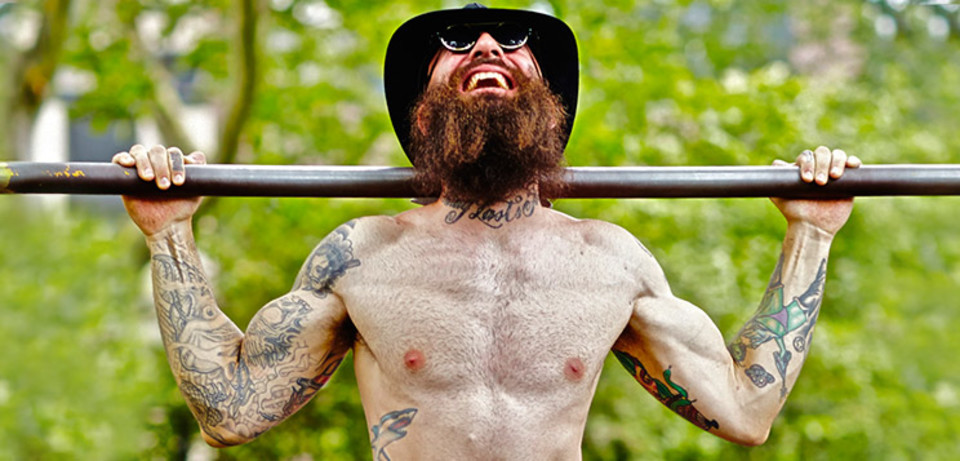The image depicts a shirtless, muscular man with a thick, bushy brown beard wearing black sunglasses and a black-brimmed hat that resembles a cowboy hat. He is lifting a metal barbell that rests across the back of his shoulders, gripping it with both hands. His flexed arms are heavily tattooed, with detailed designs that include more colorful art on one arm and predominantly black ink on the other. He also sports a neck tattoo partially obscured by his beard, and a prominent shark tattoo wrapping around the side of his torso, extending from his back. The man's chest hair is shaven but beginning to grow back. He is standing outdoors, surrounded by a blur of green trees and shrubbery, with a hint of a gray and white building in the upper left corner. His head is tilted back, mouth open, appearing either strained or in a state of exhilarated relief as he concentrates on his lift.